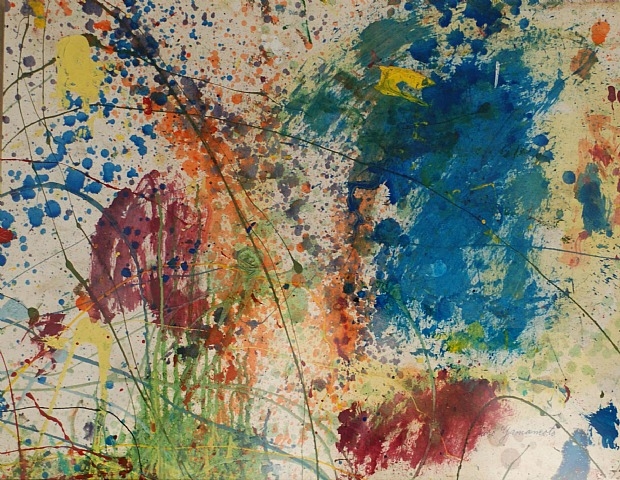This abstract painting features an energetic array of splattered and smeared paint on an off-white or light beige background, creating a chaotic yet colorful composition. On the far left side, there are blue dots resembling raindrops, accompanied by yellow blotches at the top, and beneath that, a dark orange patch. Moving from the bottom towards the right, streaks of green paint emerge, leading to a light green brushstroke that ascends slightly to the right. A prominent feature on the right side is a large blue splotch, surrounded by smaller dark blue splatters. Below this blue section, there is a mix of yellow and dark red blotches. Green strands of paint meander across the painting, adding to the random, splattered appearance. The upper right corner showcases an orange drop, followed closely by a brown drop. The entire scene is punctuated with splotches and strings of red, green, yellow, and brown paint, resembling a spirited and somewhat haphazard act of flinging paint onto the canvas.